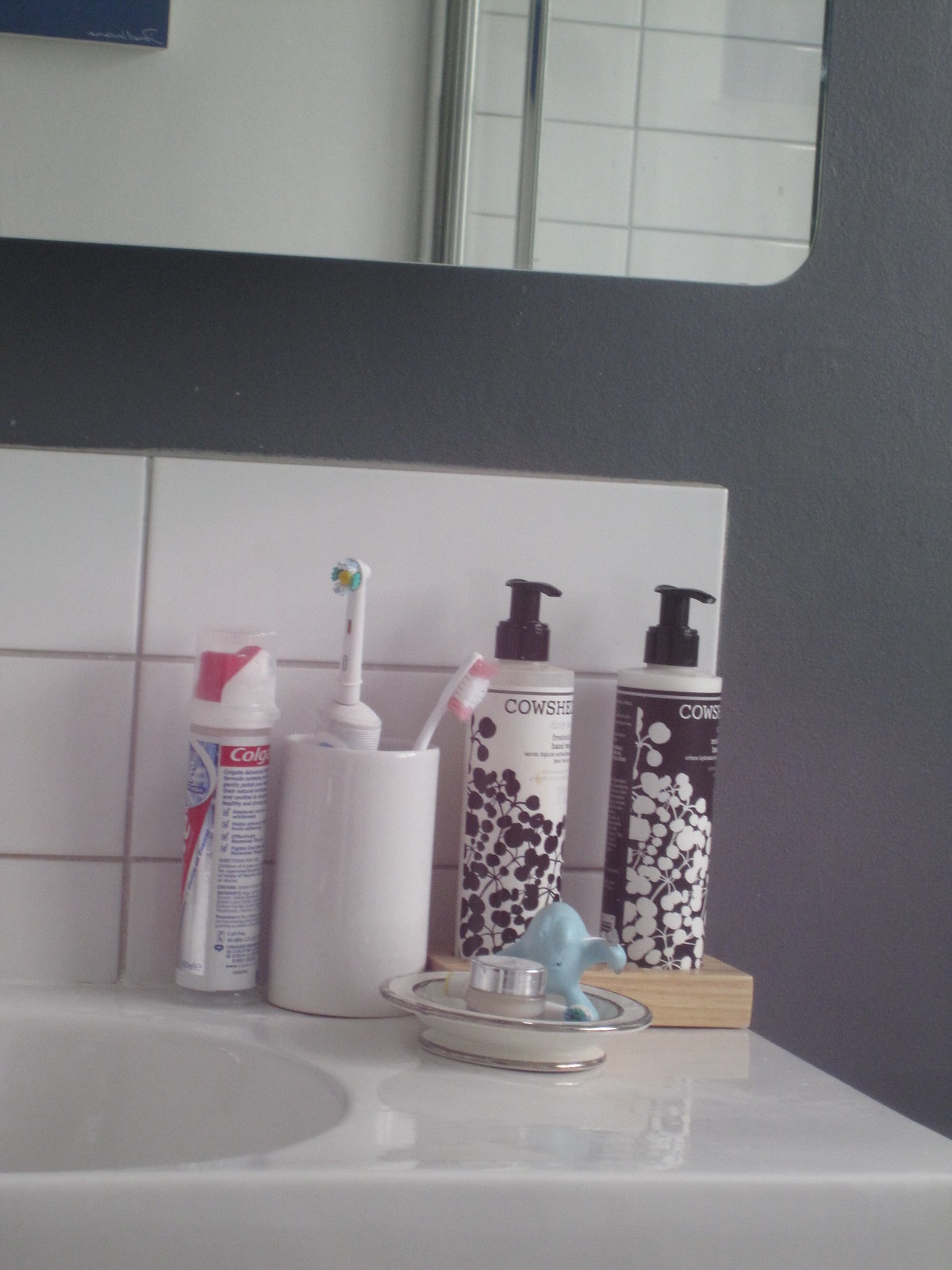A meticulously clean, white bathroom sink is visible, effortlessly blending with the flush, reflective countertop. On the right side of the sink's basin, a silver metal dish hosts a silver cylinder adorned by a small blue plastic toy, characterized by its prominent oval eyes and tiny dot-like mouth. Despite the low resolution, the toy's playful presence adds a whimsical touch.

The background is populated with various toiletry items. A notable presence is a spray can partially showing the "C-O-L-G" of the Colgate logo, equipped with a plastic cap and applicator nozzle. Nearby stands a white cylindrical toothbrush container holding a white electric toothbrush with green, yellow, and white bristles, alongside a white manual toothbrush with white bristles and pink tips.

Further to the right, two push bottles rest on a wooden rectangular stand. The bottle on the left, bearing a white label with black text, reveals partial letters "C-O-W-S-H-E," while the right bottle, sporting a black label with white text, displays "C-O-W-S." Both labels feature intricate designs incorporating plant motifs resembling vines with spherical buds.

The backdrop consists of a splash board made of sleek, rectangular white tiles, juxtaposed against a gray wall. A mirror with rounded edges occupies the upper left corner, reflecting a fragment of a blue-background painting with an indistinguishable silver signature and bar-like structures suggestive of a shower frame with matching tile-work as the splash board.

This composition captures the harmonious blend of cleanliness, functional elegance, and a touch of whimsy in a well-appointed bathroom scene.